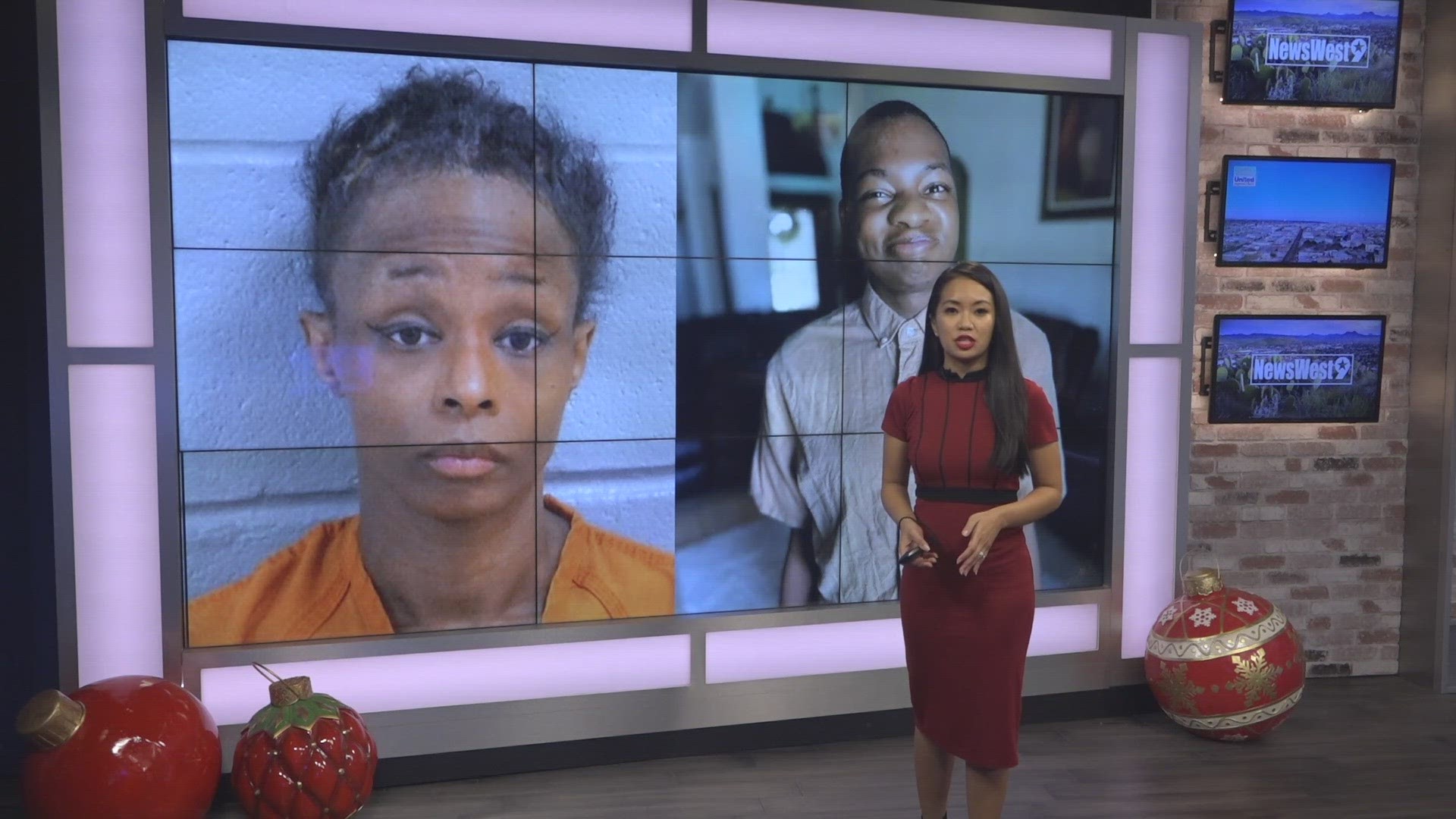In this image, a woman with long brown hair, clad in a dark red dress, appears to be delivering a report in front of a TV camera. She stands against a backdrop featuring two large projected images of young Black men. The man on the left has a somber expression and dons a yellow shirt, while the man on the right, who is slightly older, is smiling and dressed in a collared shirt. Behind her, to the right, is a large Christmas ornament, with three TV screens above it; the first and last screens display "News West 9," while the center screen shows a landscape. Additionally, two oversized red Christmas ornaments are positioned in the lower left quadrant of the scene. The overall setup suggests that she is a news reporter, possibly covering a story related to law and crime, inferred from the somber tone and the attire of the individuals in the background imagery.